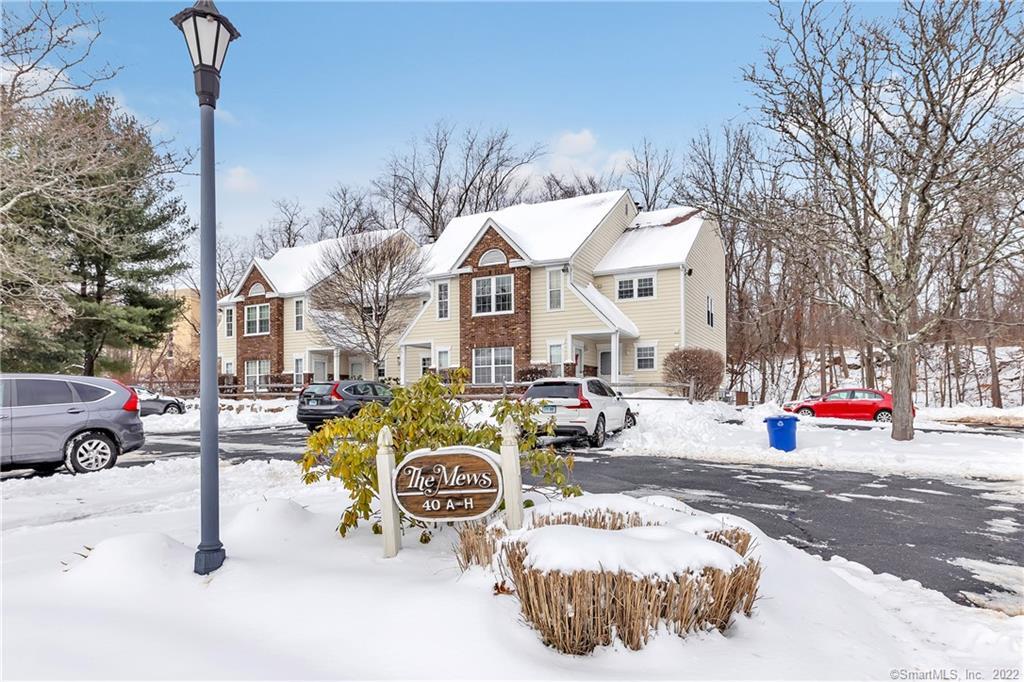The photograph depicts a winter scene of a townhouse neighborhood named "The Muse," as indicated by an oval-shaped wooden sign in the foreground held up by two white posts. The sign reads "The Muse 40A-H." In the vicinity, there is a gray lamppost to the left of the sign and a green bush beneath it, alongside another bush with brown, cut-off sticks. The image shows a corner area of a sidewalk covered in snow, leading into a roundabout and a parking lot filled with several cars including two gray SUVs, a red car, a white car, and a silver car. The townhouses in the background are three stories tall, characterized by their brick façades, triangle-shaped roofs, and large symmetrical double windows on both the first and second floors. Surrounding the buildings are leafless deciduous trees and a pine tree that still retains its leaves, all set against a backdrop of blue sky with white clouds. The photo, marked by "Smart MLS Inc. 2022" at the bottom right corner, measures approximately six inches wide and four inches high.